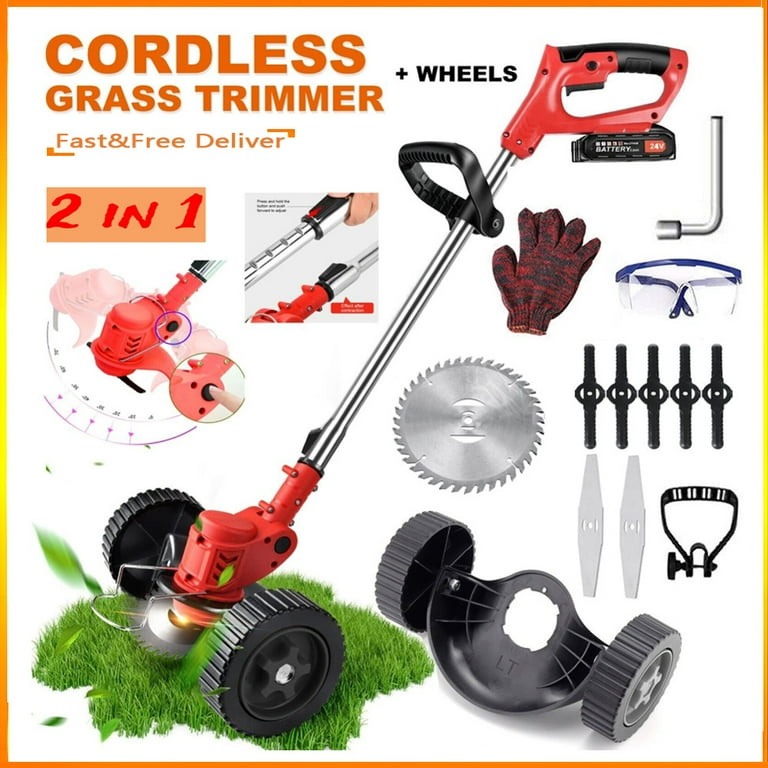This detailed advertisement for a cordless grass trimmer features a white background with a distinctive yellow and orange border that transitions from orange on the edges to yellow in the center, forming a square frame. In the top left corner, the product name "Cordless Grass Trimmer" is prominently displayed in orange font, with the text "plus wheels" in black font to the right. Below this, on an orange strip, "Fast and Free Delivery" is written in red font, emphasizing the convenience of the product. Additionally, the label "Two in One" highlights the trimmer's multifunctionality.

Dominating the advertisement is a dynamic image of the cordless grass trimmer in action, trimming a patch of grass with its head visibly spinning. To the right, multiple detailed illustrations showcase the various components and attachments of the trimmer, including additional wheels, different cutting heads, and various other parts. The accessories, which also include safety equipment like red and black gloves, and some metal and black attachments, are illustrated to provide a clear understanding of their functional diversity.

On the left-hand side, an informative illustration demonstrates how to operate the trimmer, including instructions on turning it on and off, and how to attach and detach different parts. The cordless grass trimmer itself is designed in red and black, with a sturdy black base. This ad, styled to look like it could belong to a mail-order catalog, effectively communicates the product's versatility, ease of use, and the value-added benefit of fast and free delivery.